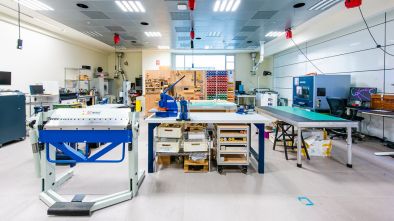The image depicts a pristine workshop, predominantly white, giving it a clean and meticulous appearance. The room is brightly lit with overhead fluorescent lights that illuminate every corner. The floor is shiny and appears as though it could be made of tile, adding to the sterile environment. The workshop is furnished with three or four desks or tables, featuring aqua blue tabletops with black borders and white legs. Various machinery apparatus are spread across the tables, hinting at a site of intricate work. In the far left, there is a row of computer terminals—approximately three—while shelves against the right wall hold other machines. Suspended from the ceiling are several red objects, possibly specialized lights essential for certain processes. The workshop also houses carts on wheels and drafting tables with stools. Electrical wiring is visible along the ceiling, adding to the industrial feel. Towards the back of the room, a large window allows natural light to filter in, contrasting with the artificial overhead lights. Nearby, a board or piece of plywood holds tools and instruments, creating a mosaic of red, blue, and green controls, further emphasizing the high-tech nature of this space.